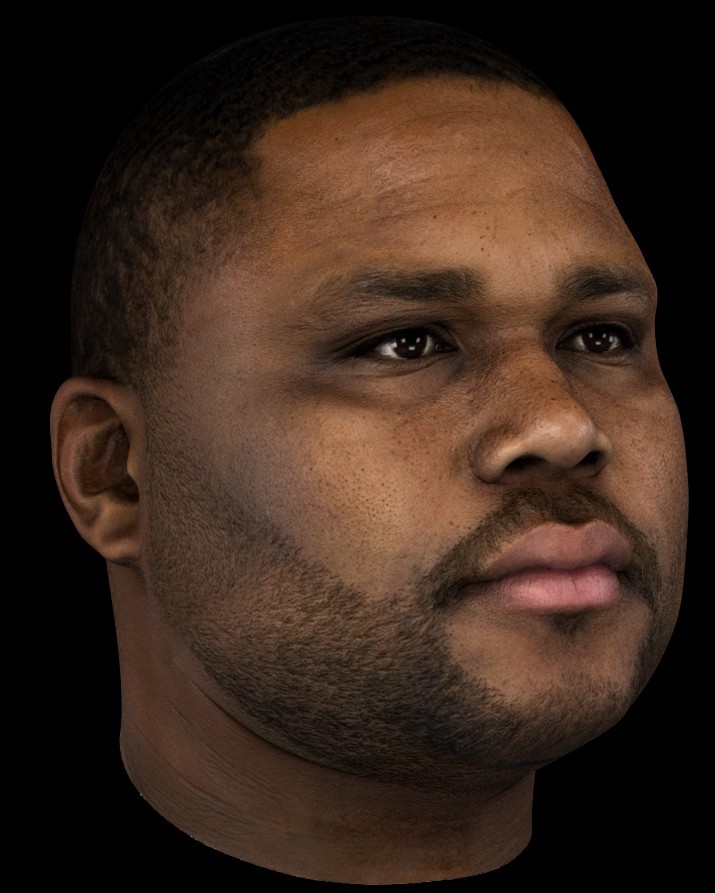This is a high-resolution photograph capturing a detailed close-up of a young black man, seemingly in his late 20s to early 30s. The image is strikingly minimalistic, set against a completely black background, which enhances the focus on the subject's facial features. He has a round, puffy face with a scruffy beard and a hint of a mustache. His short black hair frames his face as he gazes intently, slightly upwards, with a serious and neutral expression. The man's dark eyes and large lips are particularly noticeable. He is dressed in a black t-shirt with a rounded neckline, and no jewelry or accessories are visible. The photograph cuts off cleanly at his neck, further contributing to the minimalist and focused aesthetic of the composition.